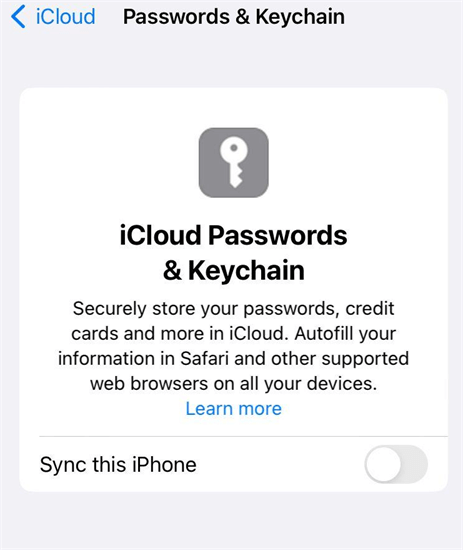This image is a screenshot displaying an interface related to iCloud and password management. The background is a very light grey, with the "iCloud" heading in blue text accompanied by a leftward blue arrow, situated in the top left corner. Centrally aligned at the top, "Passwords and Keychain" is written in black text.

Superimposed on this light grey background is a white square box. At the top of this box is a grey square with a white key icon centered inside. Below this icon, large black text states "iCloud Passwords and Keychain." Further down, in smaller black text spread across four lines, it reads: "Securely store your passwords, credit cards, and more in iCloud. Autofill your information in Safari and other supported web browsers on all your devices."

Centrally aligned beneath this text, a light blue clickable link says "Learn more." Below this link, separated by a thin horizontal grey line, the text "Sync this iPhone" appears. To the right of this, there is a slider button that is currently turned off.